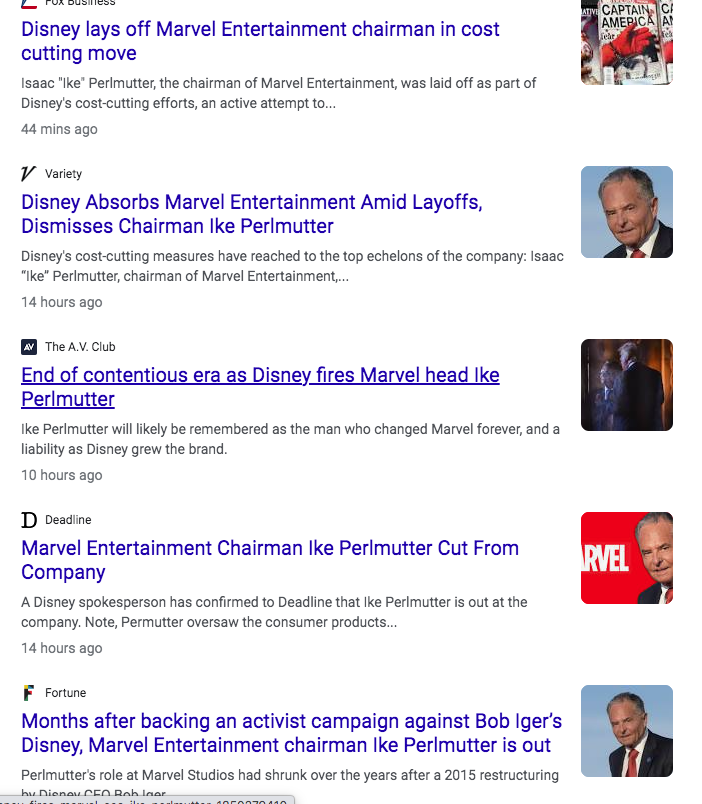**Screenshot of a Google News Page Featuring Headlines About Disney's Layoff of Marvel Entertainment Chairman**

In this screenshot, the topmost news headline is a blue, clickable link that reads: "Disney Lays Off Marvel Entertainment Chairman in Cost-Cutting Move." Accompanying this headline to the right is an image depicting Captain America wearing a handcuff. The news snippet below details that Isaac "Ike" Perlmutter, the Chairman of Marvel Entertainment, was laid off as part of Disney's cost-cutting efforts, with the phrase ending in an ellipsis. This news was posted 44 minutes ago by Fox Business.

The second headline displays a photograph of Ike Perlmutter himself and is from Variety. It states: "Disney Absorbs Marvel Entertainment Amid Layoffs, Dismisses Chairman Ike Perlmutter." The summary indicates that Disney's cost-cutting measures have reached the upper echelons of the company, affecting Perlmutter. This story was posted 14 hours ago.

There are three additional news links from the AV Club, Deadline, and Fortune, all regarding the same layoff. The AV Club's headline reads: "End of Continuous Era as Disney Fires Marvel Head Ike Perlmutter." Deadline's headline states: "Marvel Entertainment Chairman Ike Perlmutter Cut from Company." Lastly, Fortune's headline highlights: "Months After Backing an Activist Campaign Against Bob Iger’s Disney, Marvel Entertainment Chairman Ike Perlmutter is Out."